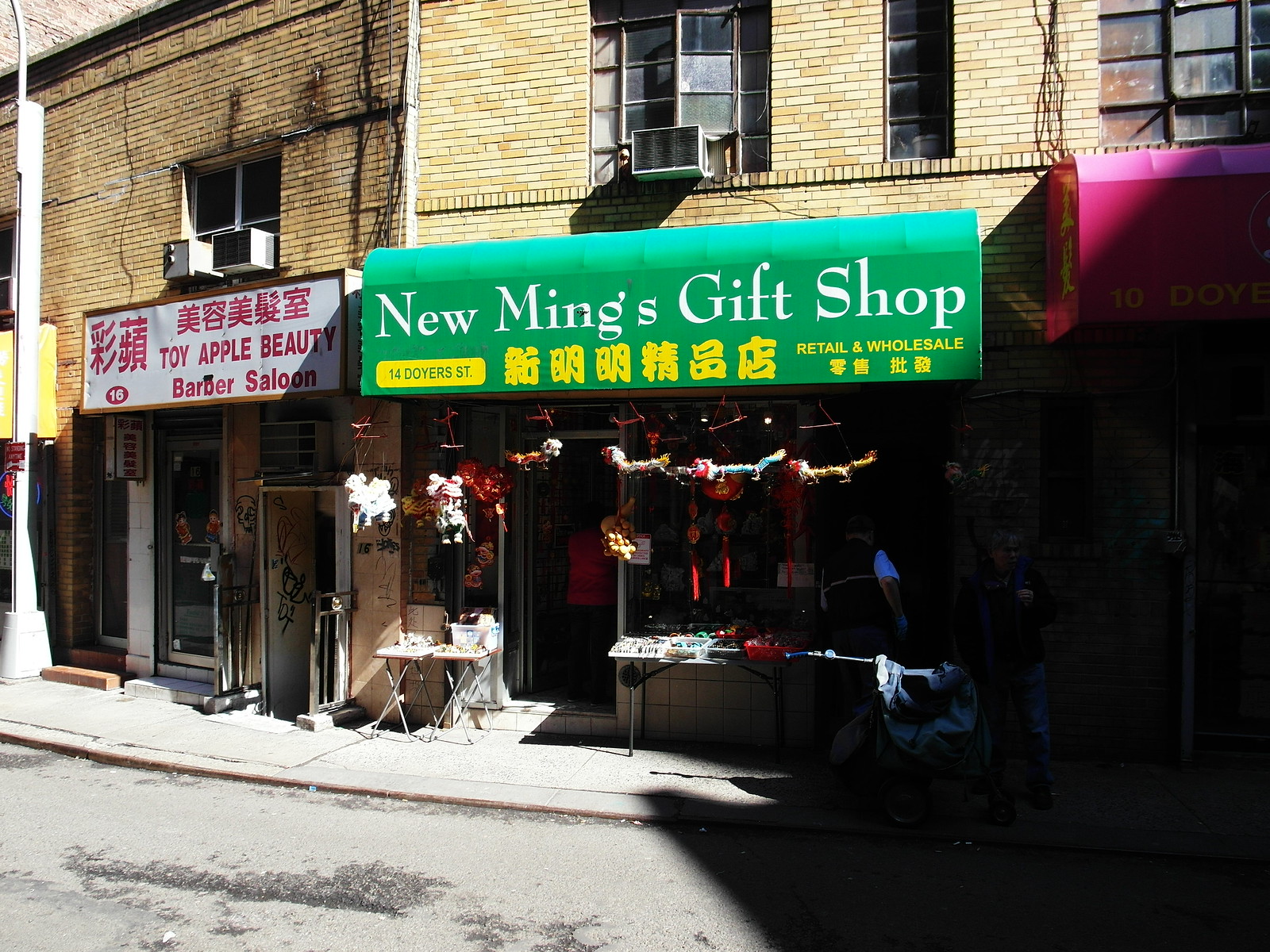This full-color daytime photograph depicts a cityscape featuring interconnected brick buildings in a bustling Asian neighborhood, possibly in Asia or an Asian district of a larger city. The buildings have two stories, with window air conditioning units jutting out from the upper-level windows. Dominating the center of the image is a storefront with a green awning that reads "New Ming's Gift Shop" in white text, accompanied by additional information in yellow text, including the address "14 Doyers Street" and Chinese characters that repeat the shop's name and details. Below the awning, there are animal-shaped decorations and Chinese dragons hanging down, adding a festive atmosphere. The shop seems well-prepared for customers, with tables set up outside on the sidewalk. To the left, another storefront with a red awning displays "Toy Apple Beauty Barber Salon" at address 16. The scene is notably devoid of people, giving it a serene, almost timeless quality.